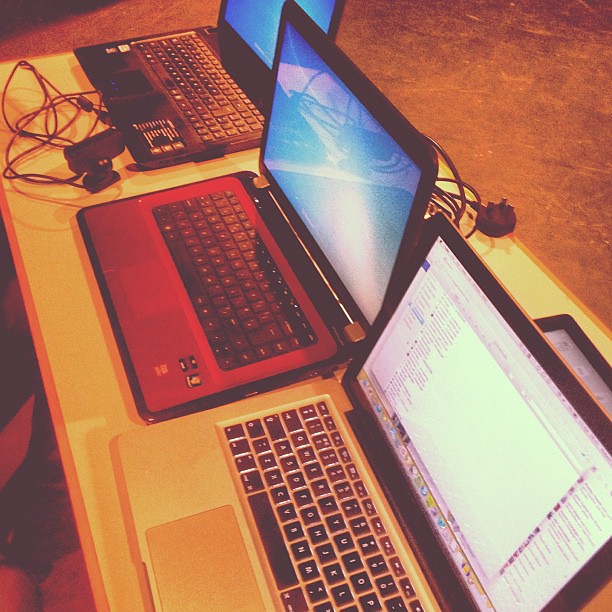The photo presents a scene with a distinct red or sepia filter, casting a warm, Mars-like hue over everything. Centered is a diagonal white table featuring three laptops, each partially visible and operational. The laptop on the far left, a silver model possibly from the early 2000s, showcases a sky scene on its blue-tinted screen and sports a red keyboard with black keys. Adjacent is an open MacBook on the right, confirmed by its operating system and interface. Its screen displays a standard file directory, alongside a yellow keyboard. The third laptop, partially visible at the top left, hints at an older design with a red keyboard yet features a modern blue screen. A pile of wires sprawls towards the left side of the table, adding a sense of clutter. The setting is grounded by a brown carpet in the background, enhancing the overall warm and vintage ambiance of the image.